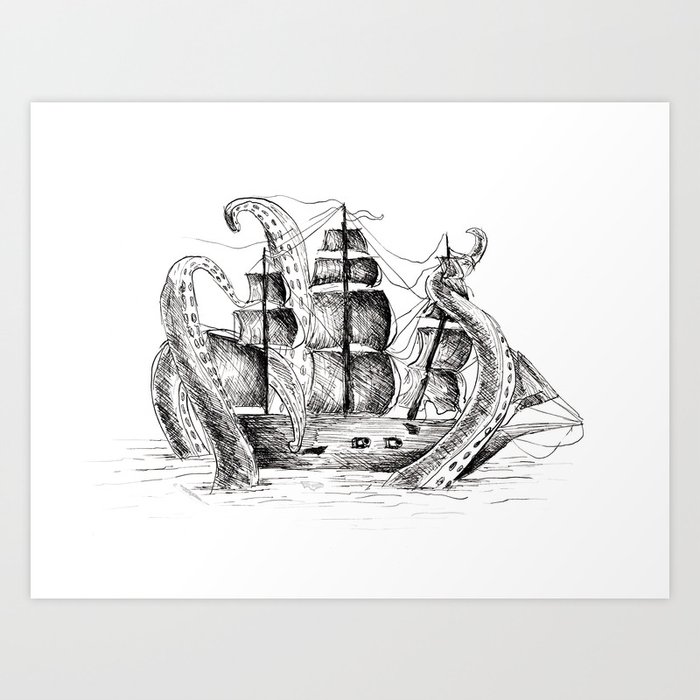This is a highly detailed black-and-white pencil sketch of a perilous maritime scene. Drawn on a white sheet of paper oriented horizontally, the background contrasts in a lilac light purple hue. Central to the artwork is a wooden boat, depicting significant wear with visible cracks and holes along its sides. The ship, featuring three spacious sails, appears caught in the midst of an attack by an immense octopus resembling the mythical kraken. Multiple massive tentacles emerge menacingly from the calm waters, one clutching the front sail tightly, while others stretch ominously over the ship's decks. The intricate entanglements of rigging and ropes add to the chaotic and doomed atmosphere, highlighting the ship's desperate struggle against its monstrous adversary.